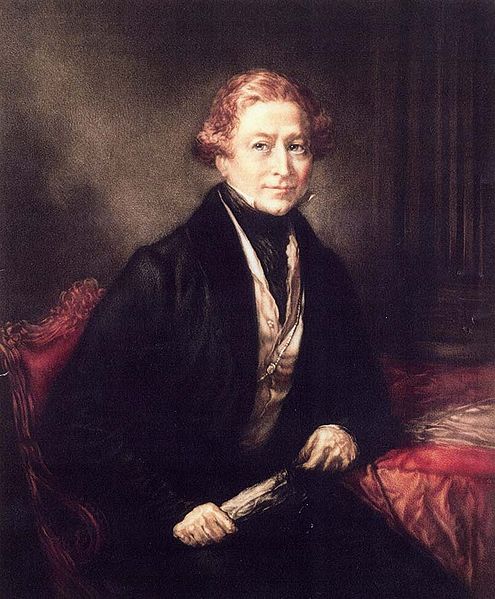The image is a historical painting of Sir Robert Peel, a distinguished Caucasian man with fairly pale skin and a slight smile on his otherwise serious face. He exudes an air of importance and nobility, emphasized by his formal attire — a long black robe over a white shirt, with a scarf tucked into his vest. His brown hair, styled to curl up near his ears, highlights his refined appearance. Sir Robert is seated on an ornate red chair with carved wood details and felt upholstery. Behind him, a red cloth serves as the backdrop. He rests his left elbow on a table with a silk tablecloth, holding a scroll in his hand. The painting, capturing the essence of the late 1700s to early 1800s, has a slightly blurred, aged look, adding to its historical charm.